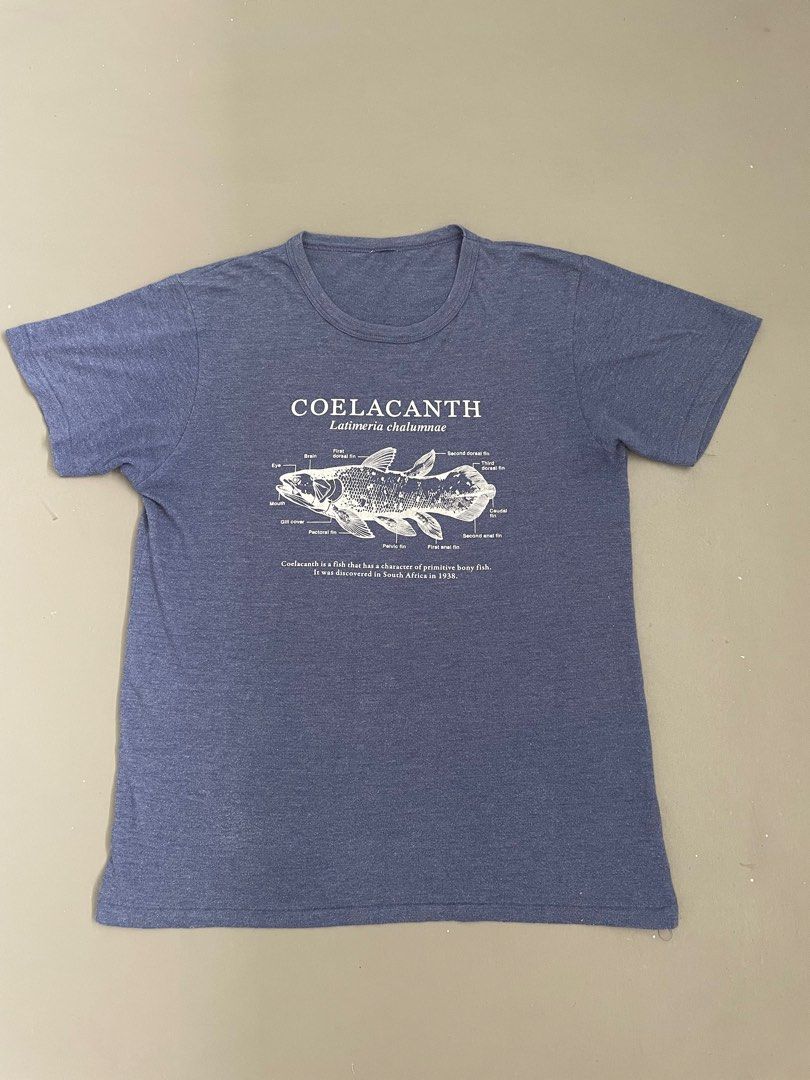This image features a photograph of a laid-out bluish-gray t-shirt on a light yellowish-gray or tan background. The t-shirt displays a detailed graphic depiction of a coelacanth fish, an ancient and still extant species, centered on the chest and spanning about three-fifths of the shirt's width. The graphic includes the fish labeled as "coelacanth," with its scientific name, "Latimeria chalumnae," beneath it. The coelacanth and the accompanying text are rendered in white against the blue-gray fabric. Tiny labels annotate parts of the fish, such as the eye, mouth, various fins (first dorsal, second dorsal, third dorsal, caudal, pelvic, pectoral), and other anatomical features. Although the text is too small to read clearly in the image, a small sentence at the bottom notes that the coelacanth is a primitive bony fish discovered in South Africa in 1938.